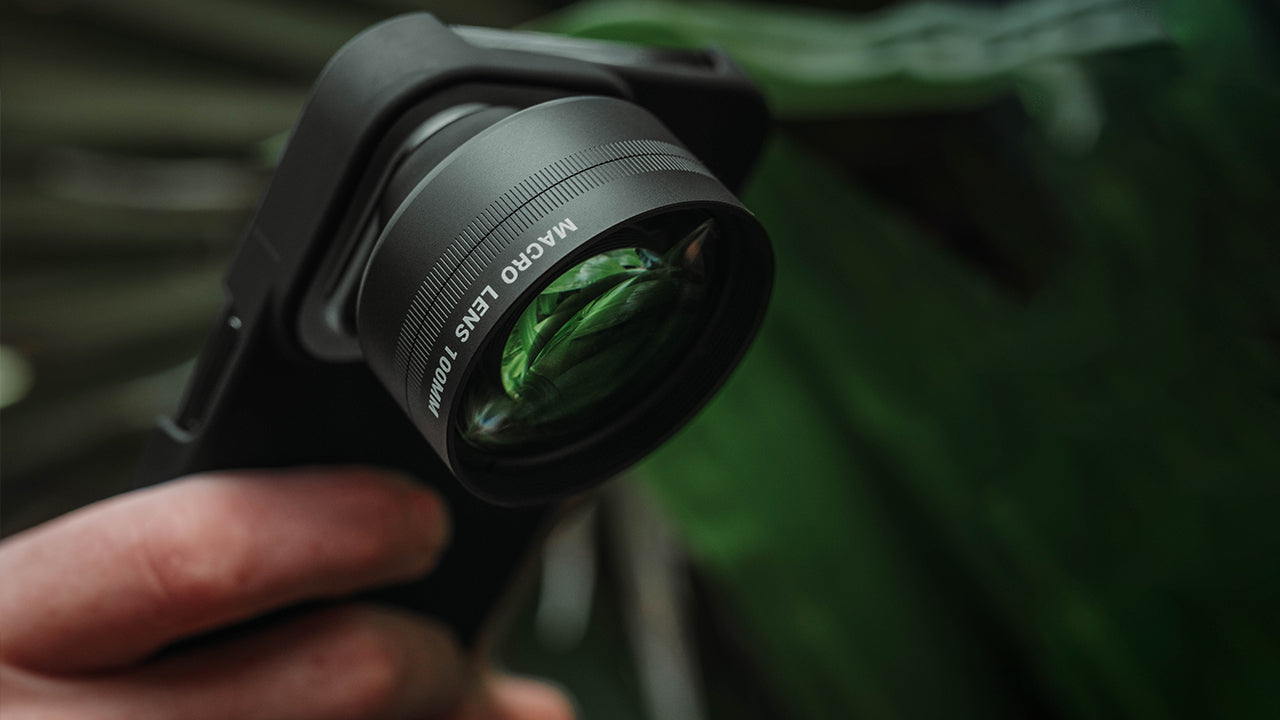In the image, a close-up showcases a black smartphone, likely an iPhone, mounted with a large, detachable macro lens. The phone is encased in a black protective cover, and a hand is visible holding it from the bottom left corner. The lens, prominently featuring the white text "Macro Lens 100mm," is cylindrical with a metal grip designed for twisting to adjust focus. The reflective surface of the lens displays the faint image of a green leaf, indicating the scene's natural surroundings. The background is a blurred mass of green foliage, underscoring that the photo was taken outdoors, capturing the essence of nature photography.